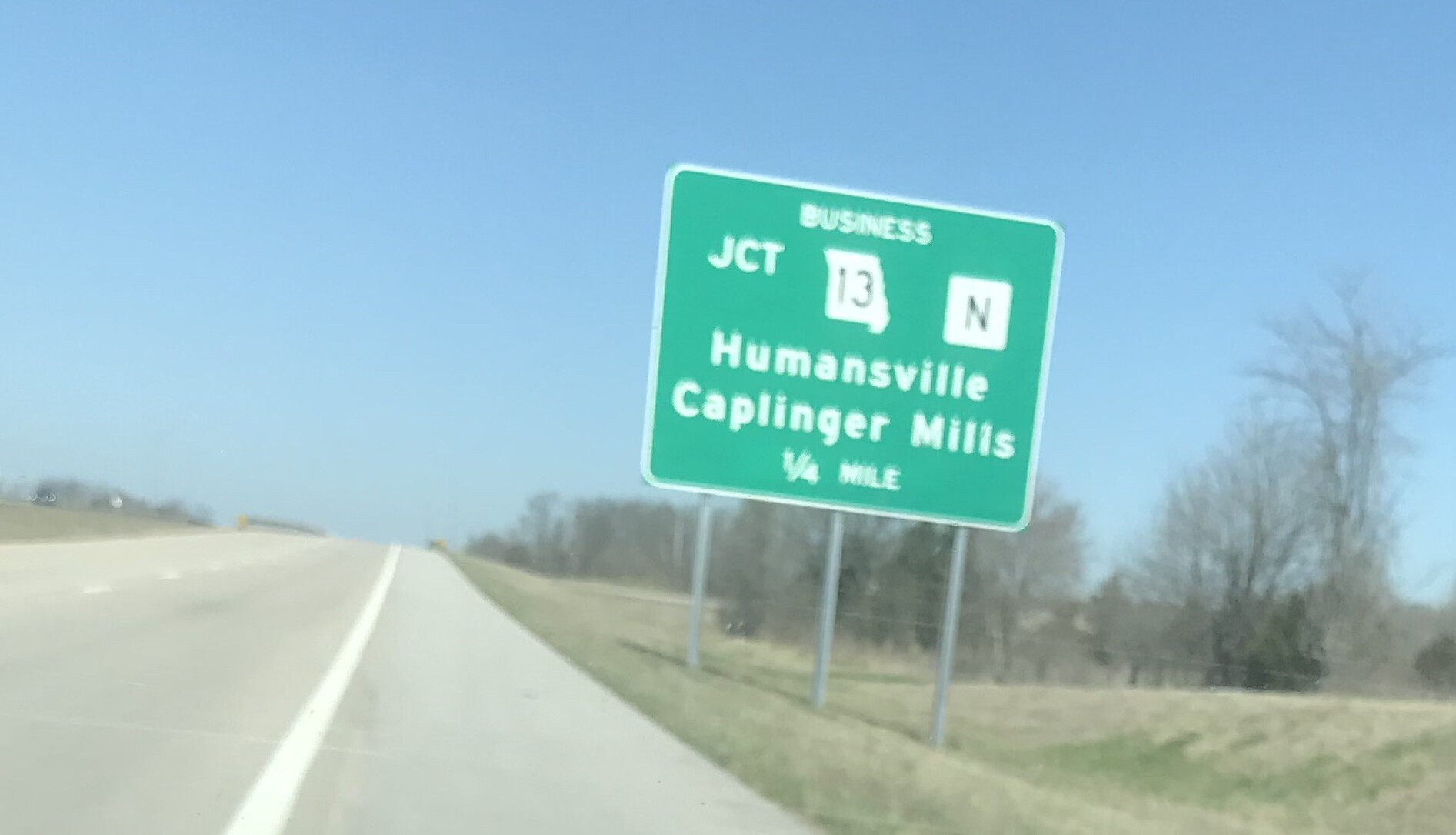The image depicts a bright, cloudless day on a seemingly deserted two-lane highway under a blue sky. The road stretches far into the distance, flanked by a solid white shoulder line on the right. A car or bike is pulled over onto this shoulder, parked past the white line as if the driver had stopped due to some issue. Surrounding the highway is a countryside scene characterized by green grass and numerous trees that are notably bare, suggesting a fall or winter setting. The focal point of the image is a large green road sign supported by three metallic poles. This sign, prominently placed for visibility, reads "Business JCT 13 Inn," with directions stating "Humansville Kaplinger Mills 1/4 mile." No buildings or other signs of population are visible, highlighting the isolation of this stretch of road in Missouri.